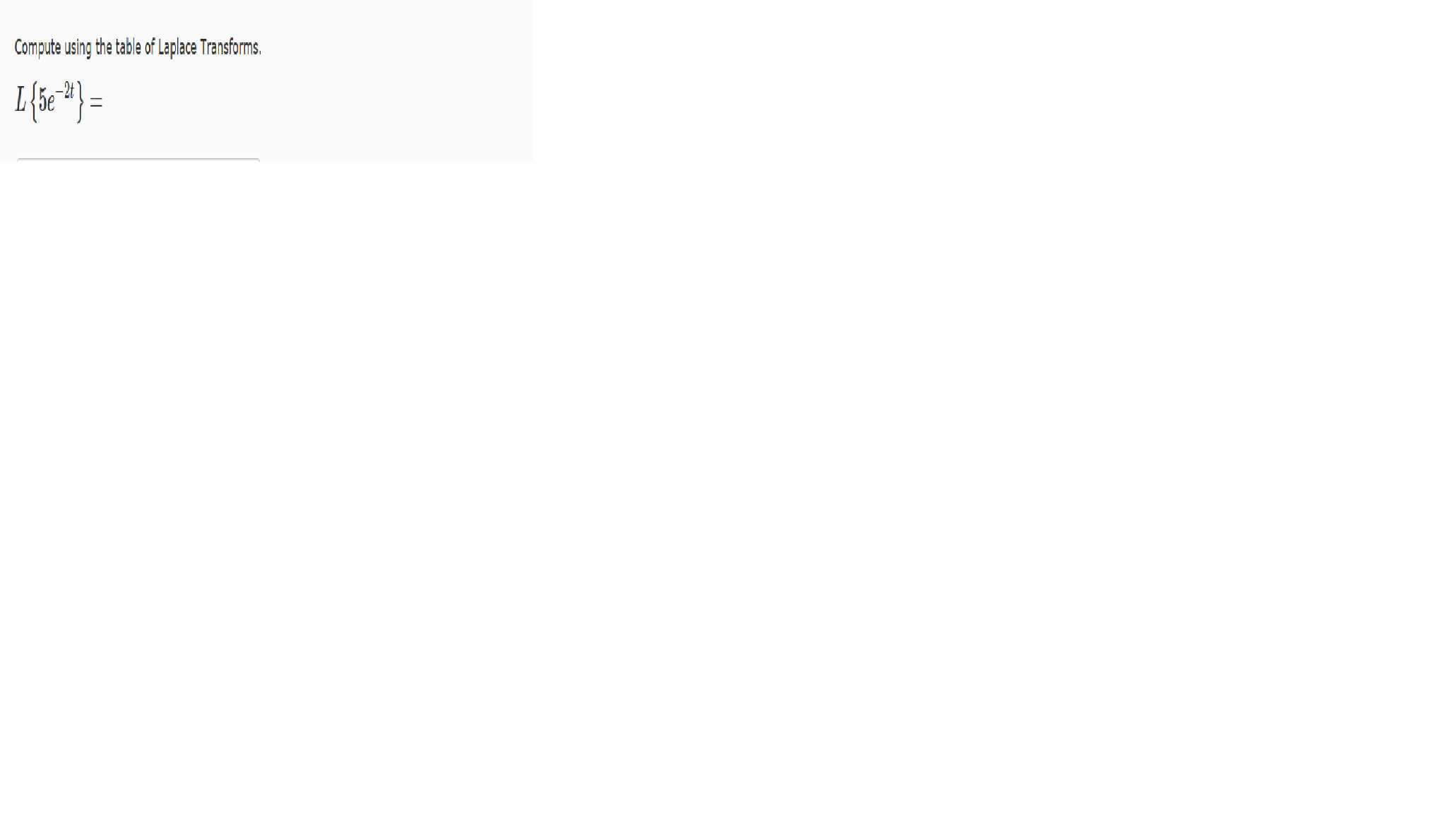This image predominantly features a blank white background. In the top left corner, there is a small, light gray rectangle with a darker gray line at its bottom left edge. Inside this rectangle, there is a single line of information in compact black text that reads, "Compute using the table of LAPLACE transforms." Beneath this text, there is a mathematical equation. The equation begins with an "L" followed by a sequence of symbols, including a number "5", an "E", and a small subscript "2", arranged between the symbols. This sequence is followed by an equal sign.